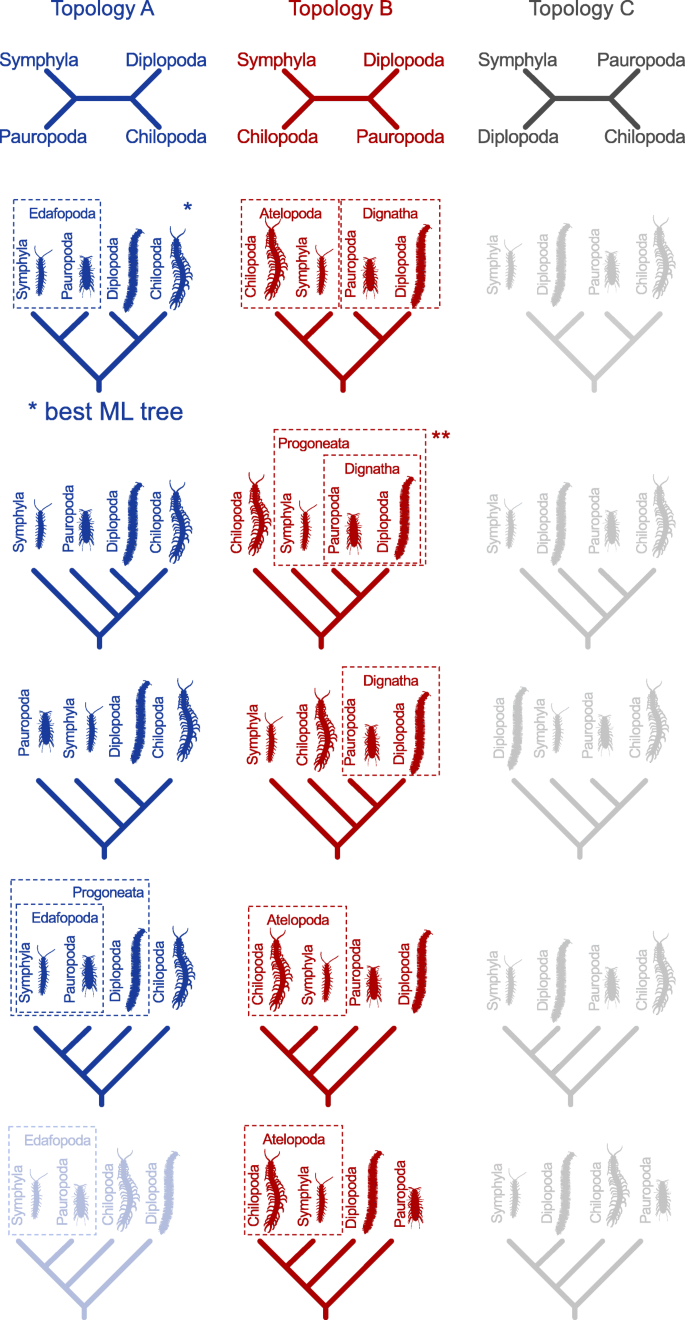The image is a tall, rectangular diagram presented in portrait layout with a white background. It consists of three vertical columns, each distinguished by color: blue on the left, red in the middle, and gray on the right. These columns are labeled "Topology A," "Topology B," and "Topology C," respectively. Each column features diagrams structured in a grid with six rows in total. 

In the top row of each column, there are X-shaped diagrams, with the lines intersecting in the center. Each section of these X's points to different classifications: Symphyla, Diplopoda, Parapoda, and Chilopoda, though their specific positions vary by column. Below the top row, subsequent rows contain detailed illustrations of various insects, accompanied by descriptive labels.

The top X-shaped diagrams are visually consistent across columns, presenting a horizontal line intersected by a V shape on each side, while the lower diagrams shift focus to individual insect representations, offering a clearer comparison of the different topological categories. This extensive visual array highlights the taxonomical differences and similarities between these insect classes across the three topologies.